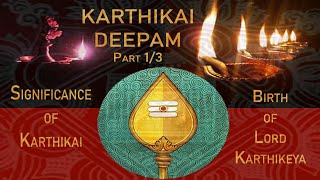This detailed image blends color photography with graphic design and illustration elements. It is oriented in landscape format with the top half featuring a black background and the bottom half in red. Dominating the upper center is gold text that reads "Karthikai Deepam," with "Part 1-3" directly below. 

On the left side, lower left, the gold text states "Significance of Karthikai," and to the right side, it mentions "Birth of Lord Karthikaia." The bottom center hosts a dark aqua elliptical shape containing a gold-colored spear tip or medallion, with the shape reminiscent of a teardrop on top of a vertical staff, also featuring a white three-stripe emblem. 

The upper left section of the image displays a photograph of an oil lamp emitting a white flame, while to the right, a row of similarly lit oil lamps can be seen against the black background, each decreasing in size toward the top right, creating a sense of perspective. Together, these elements intertwine to convey the rich cultural and religious significance of the Karthikai Deepam festival.